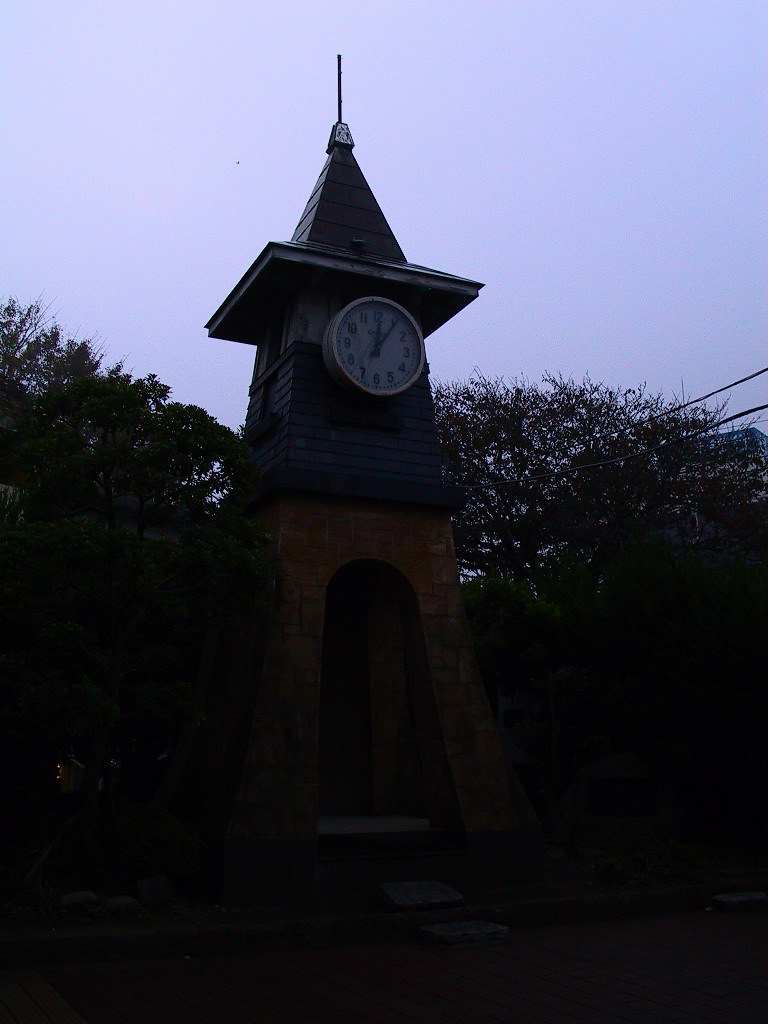In this dimly lit image taken during dusk or late evening, a towering clock structure rises prominently against a dark blue sky that lightens slightly toward the left. The clock tower itself is a multi-tiered construction, beginning with a base of brown bricks forming a large arch, possibly a doorway, extending into an open or accessible passage. Above the brick arch, the structure transitions to squared, dark gray or black bricks, separated possibly by a barely visible wooden ledge. At the midpoint of the tower sits a classic circular clock with white face and black numbers, its hands indicating the time around 12 and 1. Atop the clock, the tower narrows into a flat square section leading up to a pointed, triangular roof from which a rod extends skyward. The silhouette of tall, dark trees flanks the clock tower, and electrical lines run in the background, adding to the quaint, slightly eerie atmosphere of the scene. Stepping stones can be glimpsed leading up to the arch at the tower's base, underscoring its inviting, yet mysterious appearance.